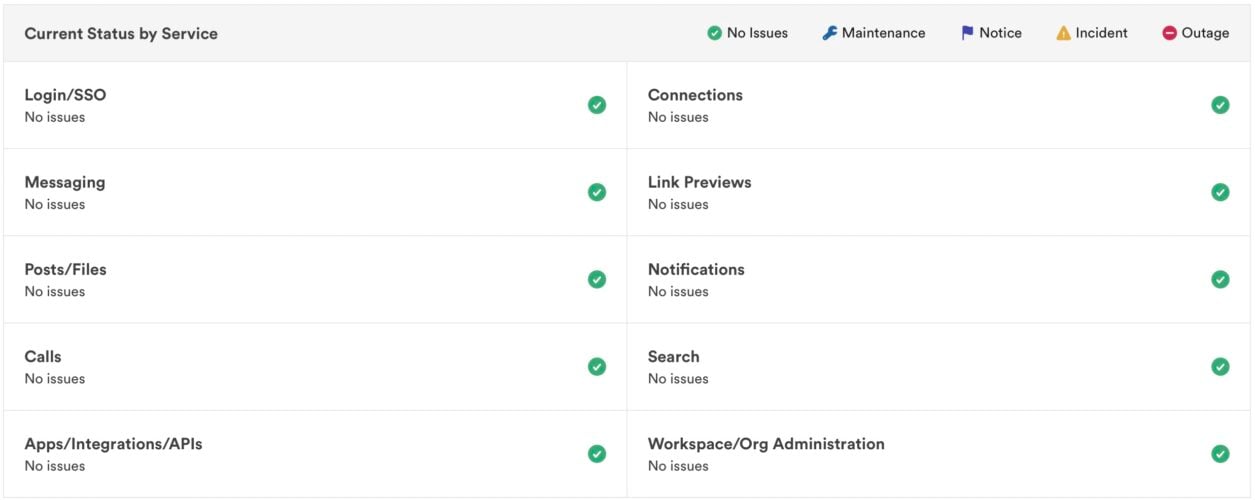This image is a screenshot from a webpage displaying service statuses. At the top, a light gray bar provides an overview with the header "Current Status by Service" in black text. On the right side of the same bar, various icons indicate different status levels: a green checkmark labeled "No Issues," a blue wrench labeled "Maintenance," a purple flag labeled "Notice," a yellow triangle labeled "Incident," and a red circle with a white line labeled "Outage."

Below the header, the page is divided into two columns listing specific services. Each service is followed by its current status:

- **Login/SSO**: No Issues (green checkmark)
- **Messaging**: No Issues (green checkmark)
- **Posts/Files**: No Issues (green checkmark)
- **Calls**: No Issues (green checkmark)
- **Apps/Integrations/APIs**: No Issues (green checkmark)
- **Connections**: No Issues (green checkmark)
- **Link Previews**: No Issues (green checkmark)
- **Notifications**: No Issues (green checkmark)
- **Search**: No Issues (green checkmark)
- **Workplace/Org Administration**: No Issues (green checkmark)

Each status is marked with a green checkmark, indicating that all systems are functioning normally without any reported issues.